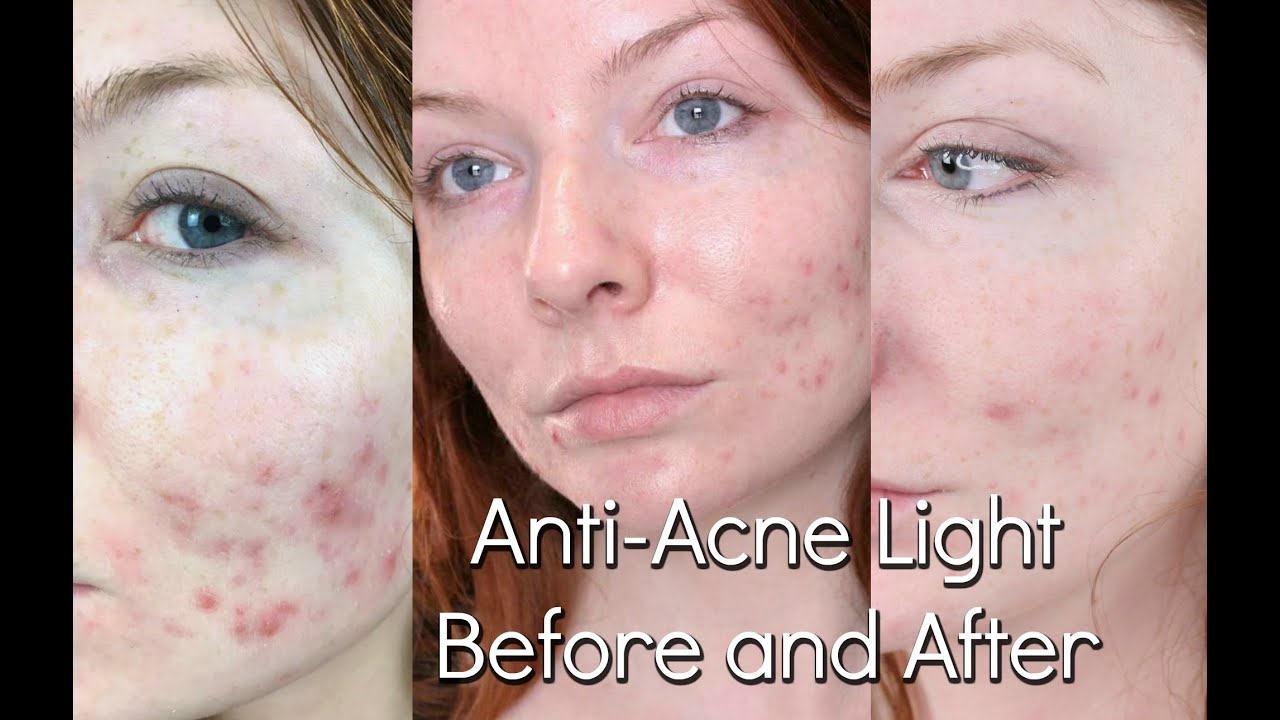This image showcases a before-and-after progression of anti-acne treatment through three slides. The first slide displays a girl's pale face, with visible acne concentrated on her cheek. The second slide shows a more encompassing view of her face, where the acne appears significantly reduced in severity, though her overall skin tone is notably different from the first slide. The third slide offers a partial view of her face, revealing a cheek with almost no acne, although her skin tone is somewhat paler compared to the second slide, yet not as pale as in the first. Each slide is labeled accordingly to highlight the stages of improvement, suggesting the efficacy of the treatment, though there is some ambiguity about whether the images depict the same person across all three slides due to variations in skin tone.